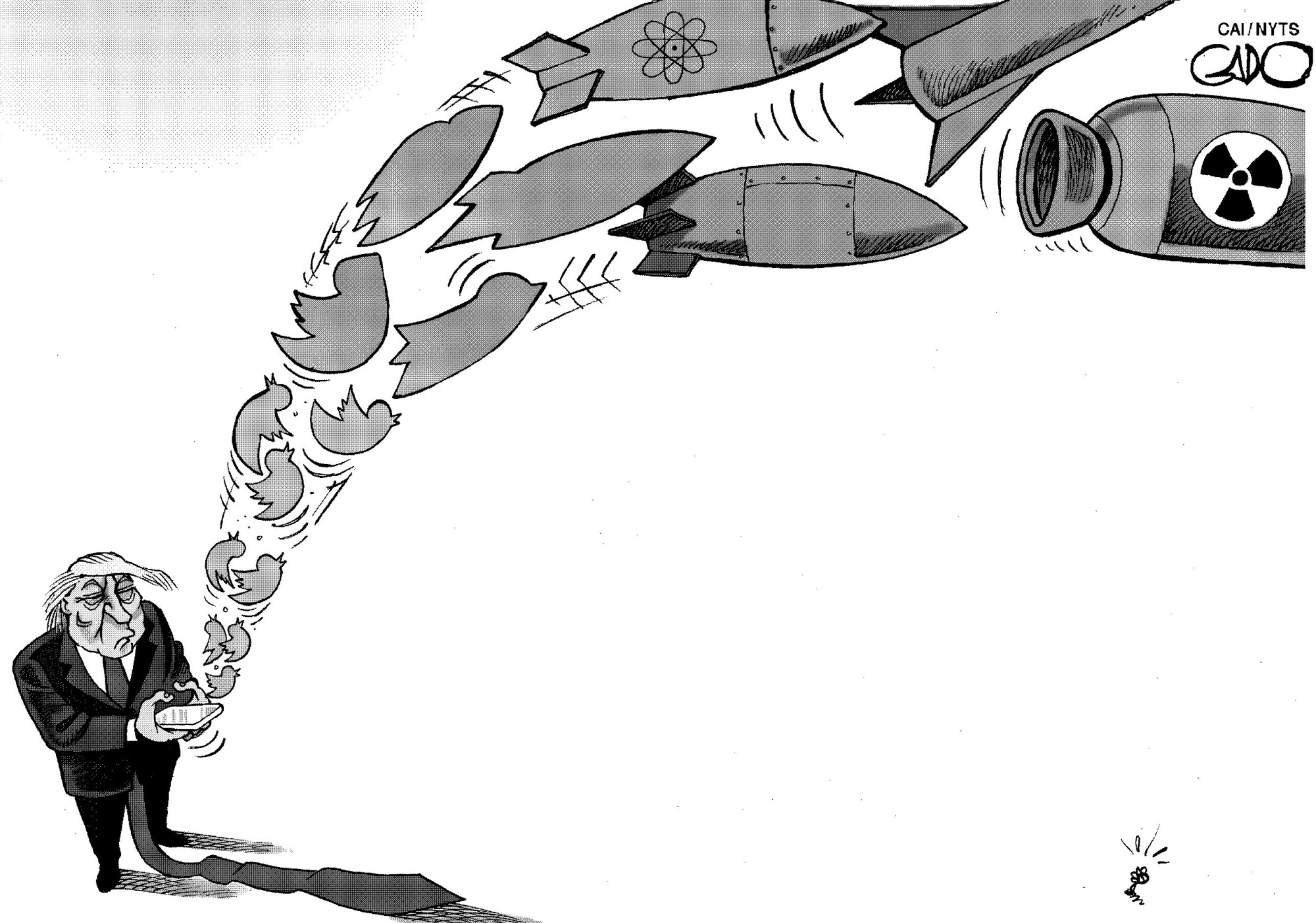This black and white political cartoon, rendered in grayscale, features a depiction of Donald Trump in the bottom left corner. The artist has paid considerable attention to his distinct hair and an exaggeratedly long tie that extends down to the floor. Trump is portrayed with a grumpy, bored facial expression and is wearing a black suit, accompanied by black pants and shoes. He is holding a smartphone from which a series of Twitter logo birds are emanating. These birds arc from the bottom left towards the top right of the image, gradually transforming into bombs and missiles, some marked with poison symbols and one with a nuclear symbol. The top left corner features a patterned background, while the top right corner includes a partially faded signature of the artist, with what appears to be letters spelling out a name or moniker. The cartoon, styled in a manner reminiscent of newspaper political cartoons, effectively critiques how the content shared on social media can escalate into violent actions.